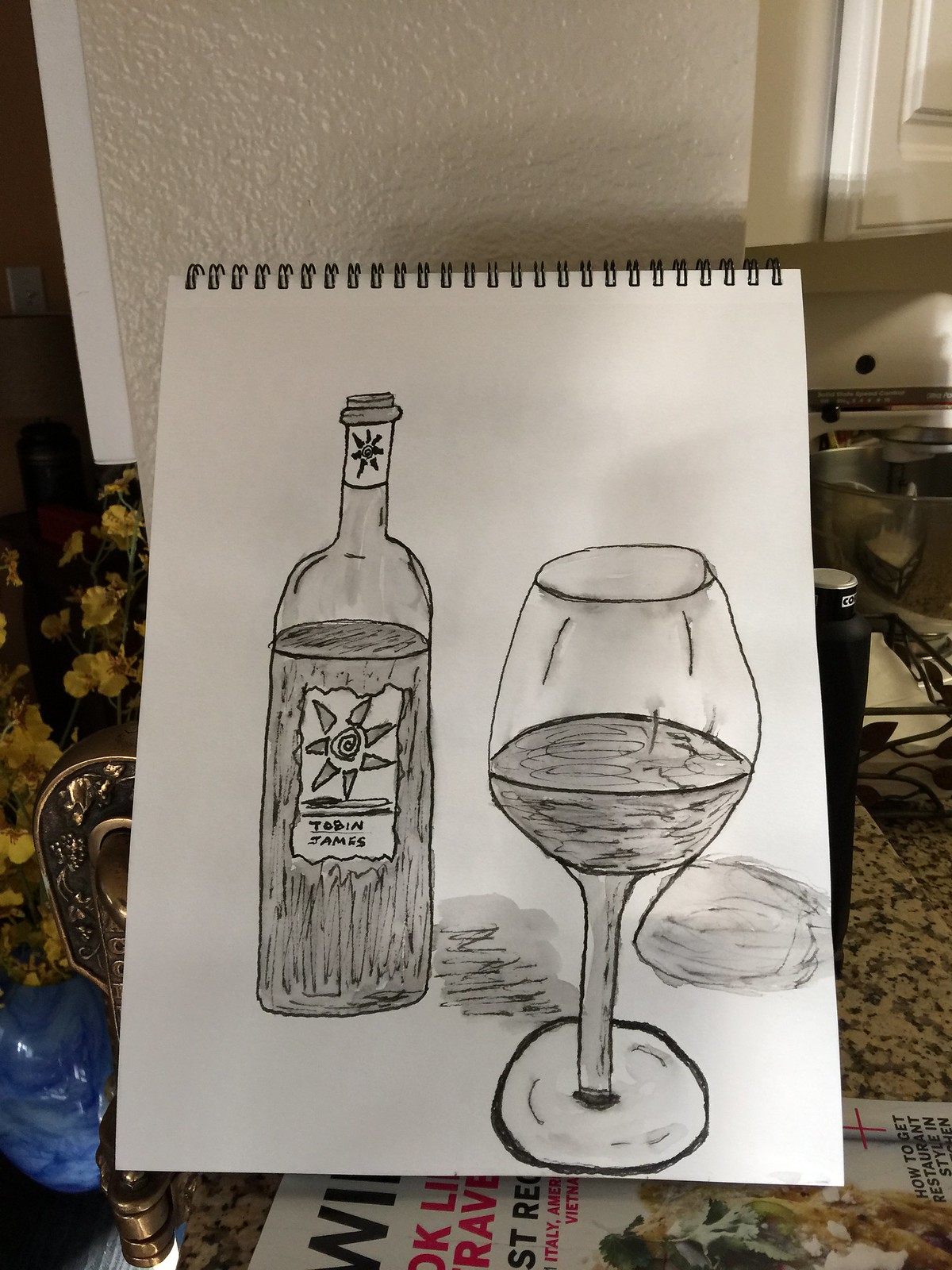The color photograph captures an intricate scene within what seems to be a kitchen. Central to the image is a sketchbook, positioned upright, bound at the top with white wire spirals. The prominently displayed sketch, done in black pen or marker, features a bottle of Tobin James wine identifiable by its label adorned with a distinctive sun motif both on the bottle's body and near the cork. Adjacent to the bottle, on the right, a wine glass, partially filled, is drawn slightly closer to the viewer, casting a subtle shadow. The background reveals a textured white wall, a granite countertop, and various elements including flowers, metal hardware, and scattered papers, enhancing the lived-in ambiance of the kitchen setting. The sketchbook's positioning hints at a casual yet cluttered environment, fostering an intimate glimpse into the blend of artistry and everyday life.